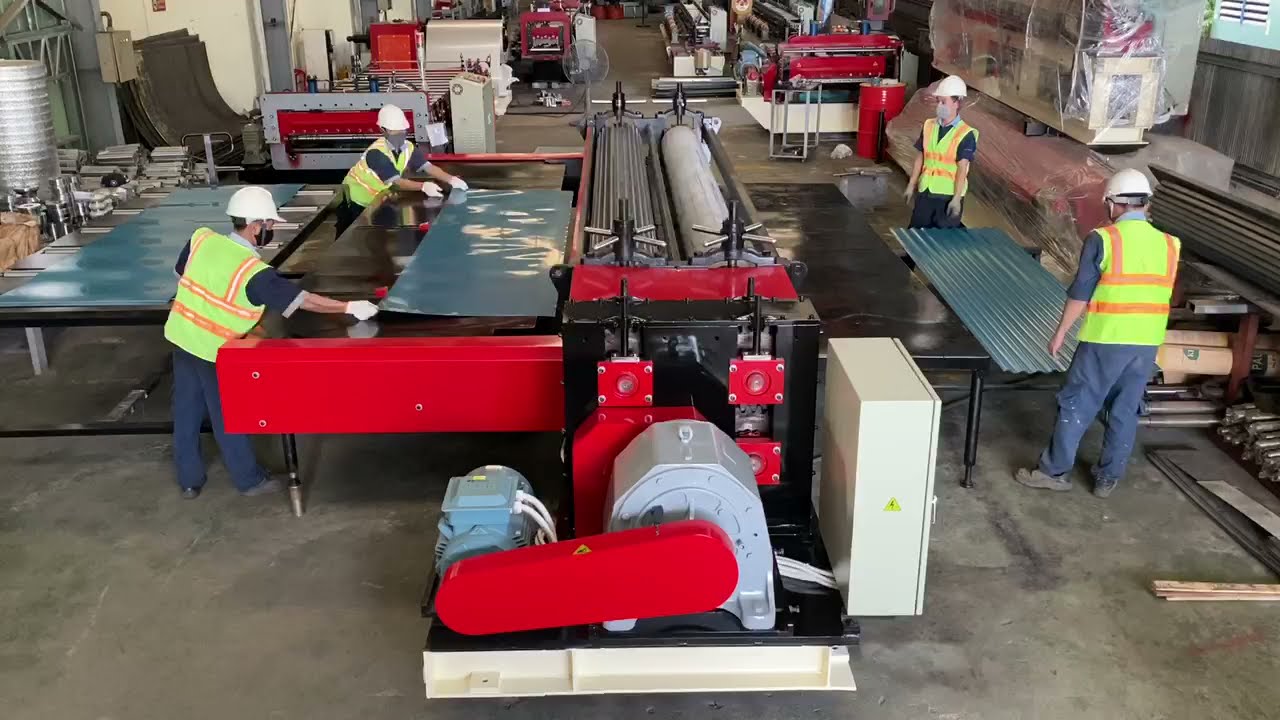The image depicts the interior of a spacious and professional factory assembly room. Central to the scene is a large and colorful metalworking machine, predominantly black and red with some white and grey components. Four workers, each wearing neon yellow reflective safety vests, white hard hats, and brown uniforms, are engaged with the machine. Two men on the left are feeding a thin sheet of metal into the machine, while the other two men on the right handle the corrugated metal sheet as it exits. The factory space contains various other machines scattered in the background, emphasizing an organized yet bustling industrial environment. Surrounding the main action are additional materials and supplies, suggesting a well-equipped manufacturing facility focused on safety and efficiency.